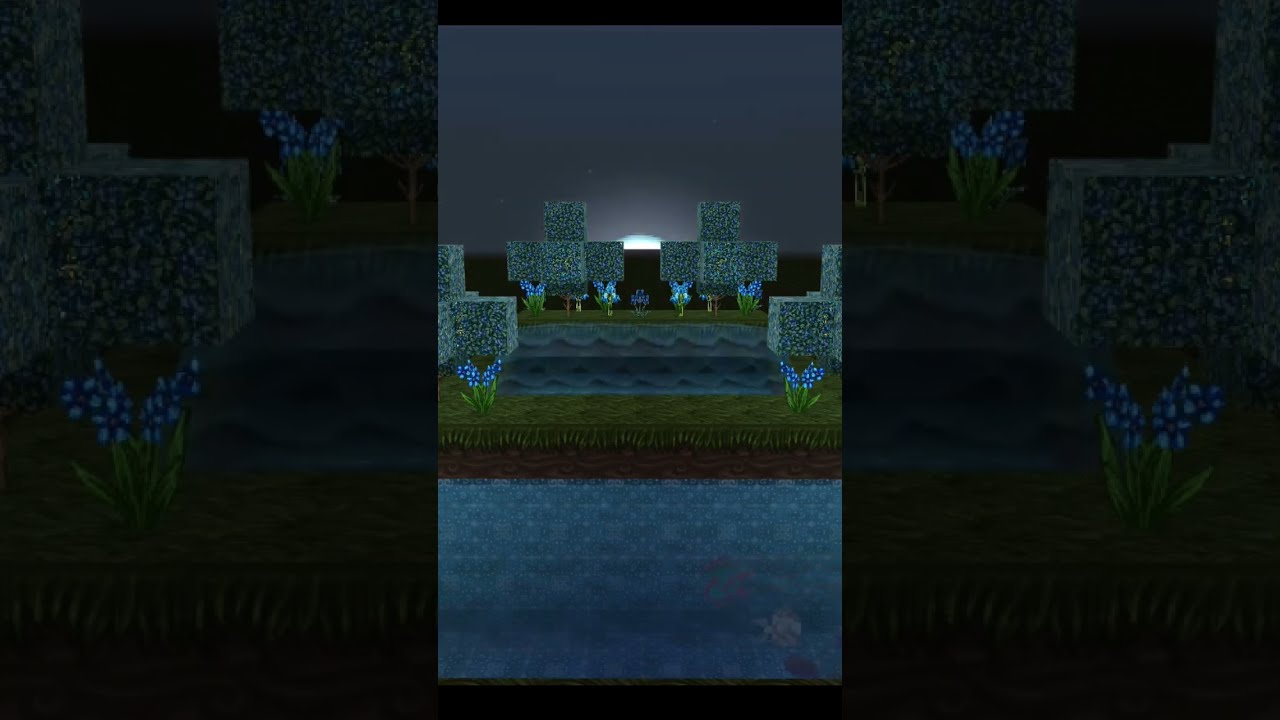This image is a detailed and dark computerized graphic from the video game Minecraft. It portrays a rectangular scene captured at dusk with the setting sun casting a charcoal hue over a meticulously designed garden. The central vertical rectangle, reminiscent of Minecraft's iconic blocky aesthetic, shows green grass blocks adorned with small plants and distinctive blue flowers set amid symmetrical stone blocks. A small portion of the moon peeks out from behind neatly trimmed bushes, casting a faint white glow. The left and right sections of the image blur into close-ups, mirroring the central scene's elements but with more indistinct outlines. These areas emphasize the transitions, drawing attention to the horizontal composition. The scene is set against a dim gray sky, enhancing the overall silhouette effect and highlighting the serene, twilight atmosphere of the pixelated garden.